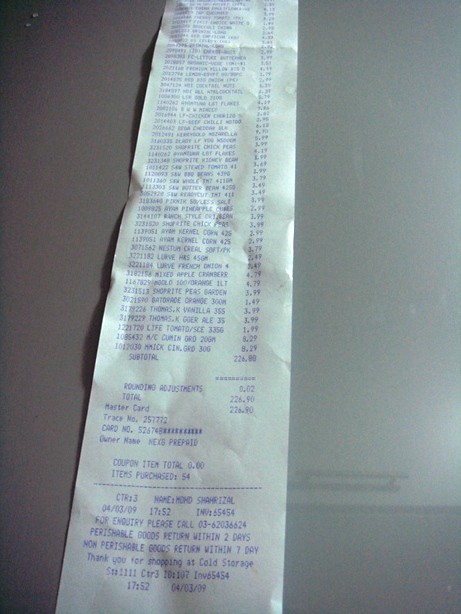This image displays a very long receipt lying on a plain, dark, grey background, possibly a table or desk. The receipt is from a store called Cold Storage, featuring a lengthy list of 54 items purchased, reflecting a substantial shopping trip. Some identifiable items include cumin, and potentially turmeric, along with mentions of tomato, kernel corn, mixed apple, and cranberry. The total amount spent is visible as $226.90, paid using a MasterCard. Although the image is blurry and the text is small, it includes key details such as a transaction date from 2009 at 17:52, a non-USA phone number for inquiries, coupon item totals, and standard return policies for both perishable (within two days) and non-perishable goods (within seven days). The receipt also shows the owner's card information, largely redacted, but marked as prepaid.